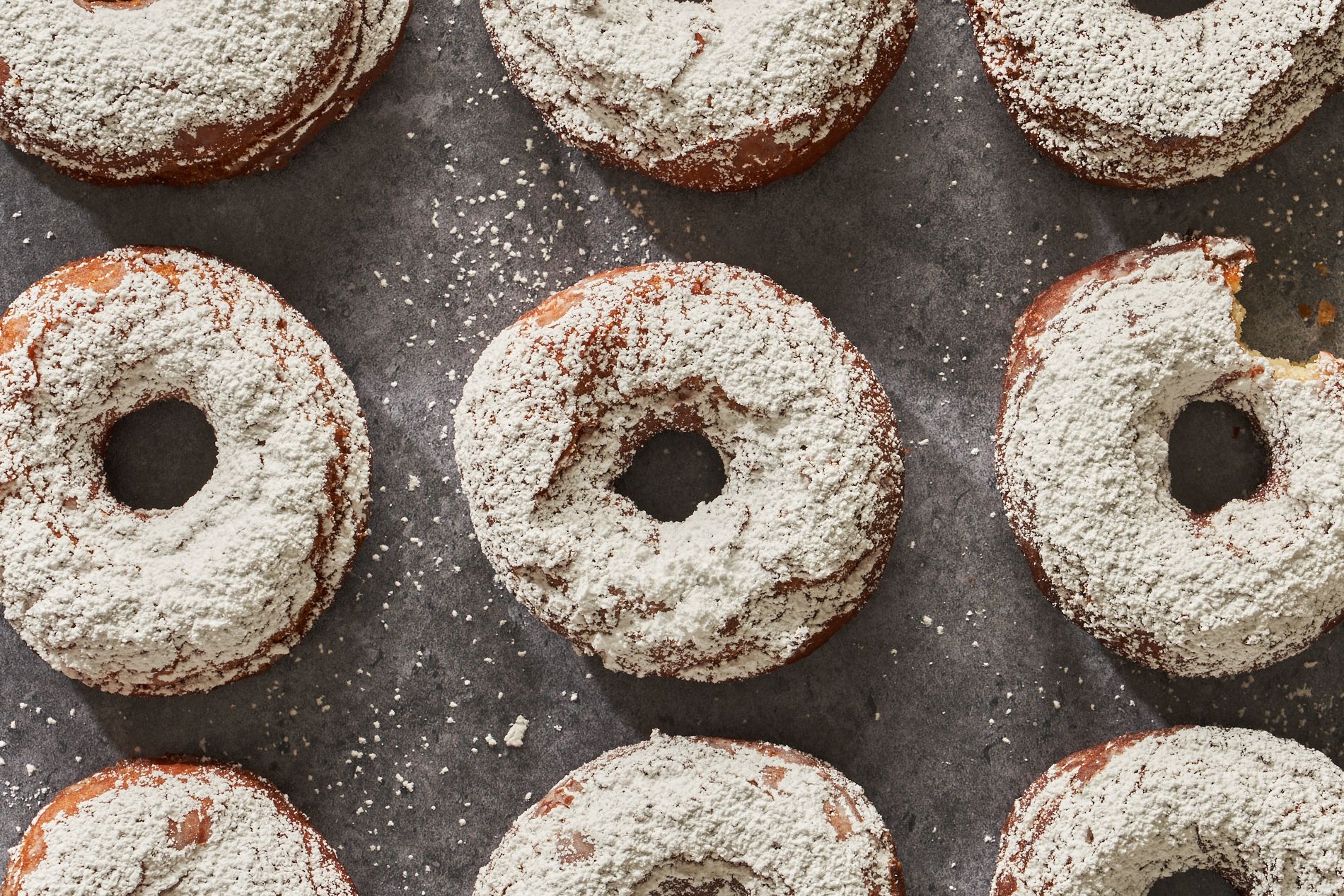The photograph showcases nine plain doughnuts arranged in three distinct rows against a gray, speckled background. The top and bottom rows each display the lower and upper halves of three doughnuts, respectively, while the middle row features three fully visible doughnuts. Each doughnut is round with a central hole and coated generously in powdered sugar. The background, dusted with specks of powdered sugar, hints at a recent dusting or decoration process. Particularly notable in the middle row, the doughnut on the far right has a visible bite taken out of it. The color palette of the image features shades of gray, white, and hints of tan from the doughnuts themselves. This vibrant and detailed arrangement, with its clean and appealing presentation, could easily serve as an advertisement for a bakery.